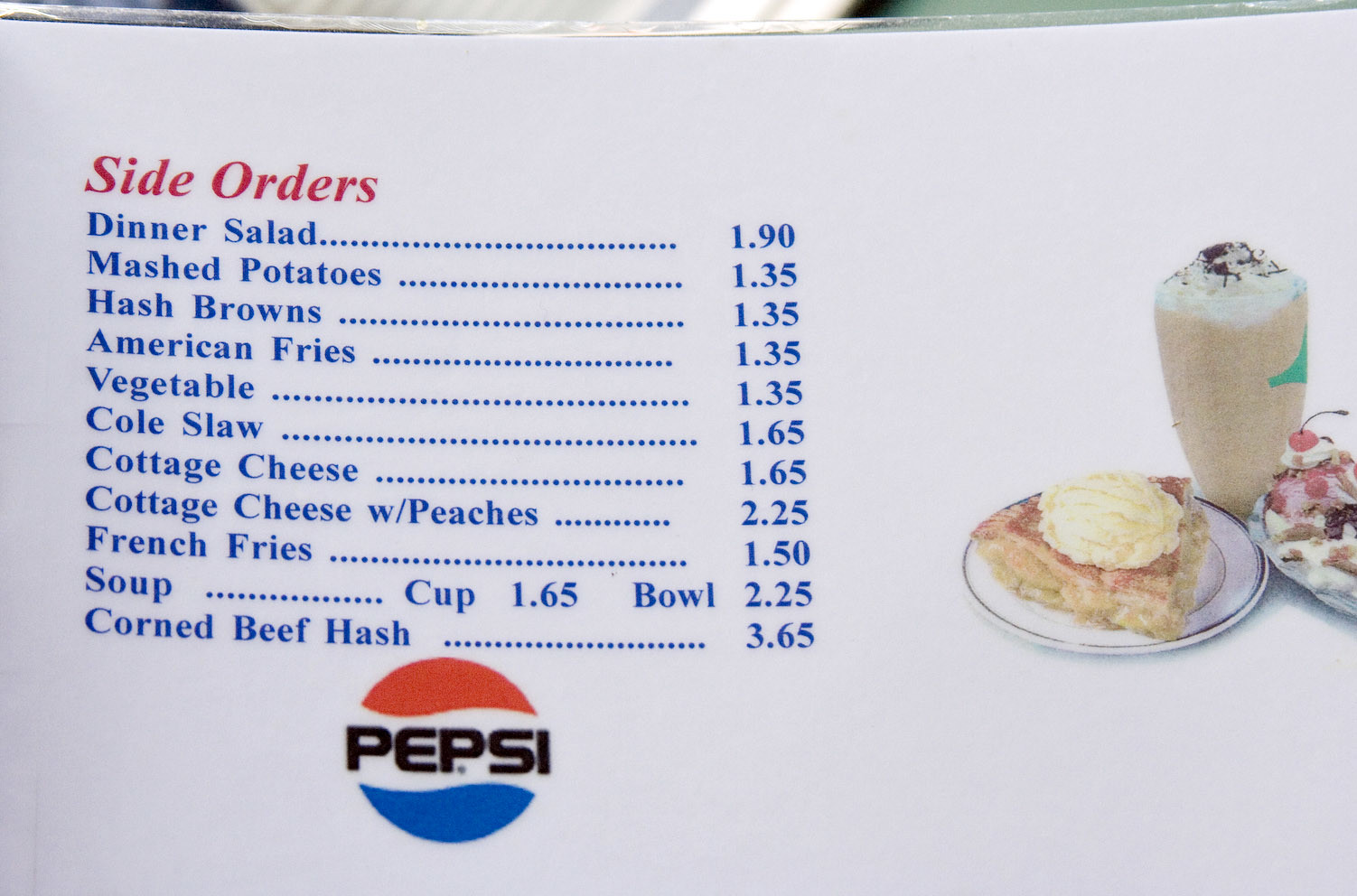The image displays a white menu featuring a "Side Orders" section in red syrup-like typography. The menu lists items and their prices: Dinner Salad - $1.90, Mashed Potatoes - $1.35, Hash Browns - $1.35, American Fries - $1.35, Vegetable - $1.35, Coleslaw - $1.65, Cottage Cheese - $1.65, Cottage Cheese with Peaches - $2.25, French Fries - $1.50, Soup (cup) - $1.65, Soup (bowl) - $2.25, and Corned Beef Hash - $3.65. To the right of the menu, a tan milkshake topped with whipped cream and chocolate shavings is visible, alongside a slice of apple pie with a scoop of vanilla ice cream and part of an ice cream sundae. The top edge of the menu and image are also visible. At the bottom right corner of the menu, the logo of Pepsi is prominently displayed, characterized by a red, white, and blue circular design with the brand name "PEPSI" in all capital letters and a white wave cutting through the circle. The food images appear slightly faded and are not very vibrant or large relative to the menu's size.